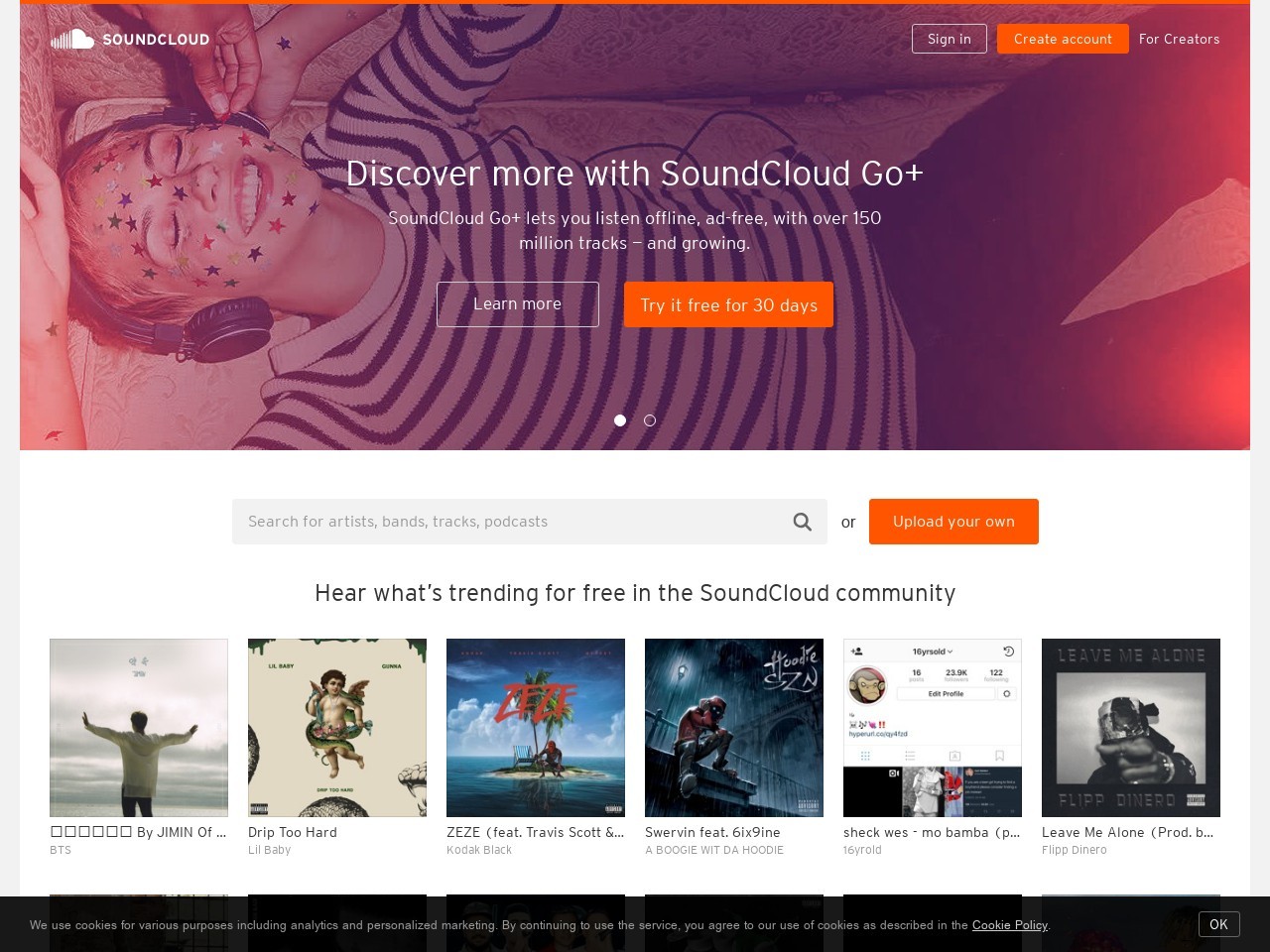The webpage showcases the SoundCloud platform, featuring the prominent SoundCloud logo—a stylized cloud with the word "SoundCloud" next to it—situated in the top left corner. Dominating the top portion of the page is a large banner. The banner illustrates a person lounging comfortably, either on their side or on a couch, wearing headphones and smiling with their eyes closed. The individual is adorned in a striped shirt and pants, and their face and arm are embellished with vibrant, multicolored stars.

To the right of the SoundCloud logo at the top, there are navigational links labeled "Sign In," "Create Account," and "For Creators." Beneath these options, still within the banner, is a promotional message: "Discover More with SoundCloud Go Plus." This service is advertised as allowing users to listen offline and ad-free to a library that boasts over 150 million tracks and counting. Below this message are two call-to-action buttons: one labeled "Learn More," and the other, highlighted in orange, reads "Try It For Free For 30 Days."

Continuing down, there is a search bar that prompts users with "Search For Artists, Bands, Tracks, Podcasts" and an adjacent option to "Upload Your Own." Below the search bar, a heading announces, "Here's What's Trending For Free in the SoundCloud Community." Following this, the page displays a series of album artwork, featuring artists like Jimin, Drip Too Hard, Jazay, Swervin' feat. Sheck Wes, and Leave Me Alone.